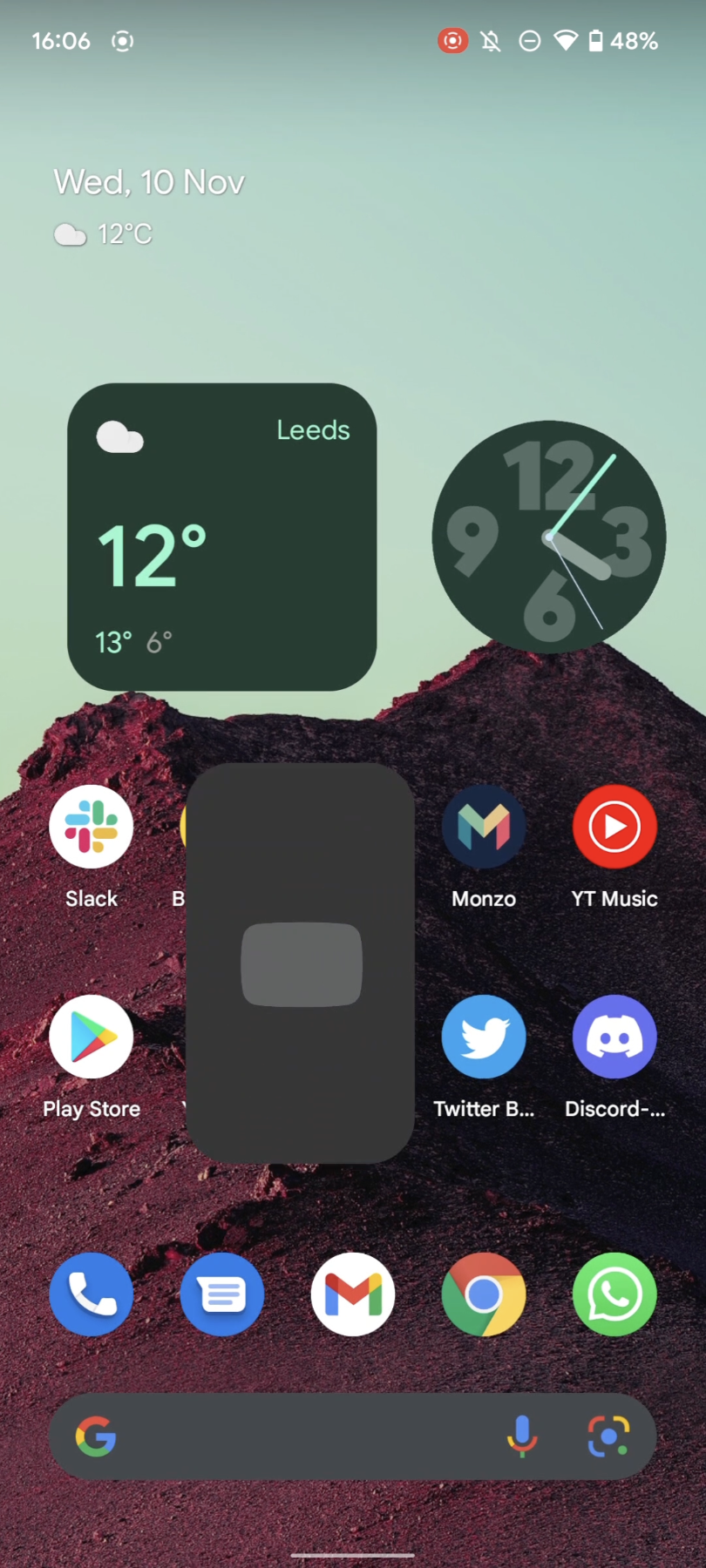In the image, we observe the home screen of an Android smartphone. The time displayed at the top left corner of the screen reads 16:06. Adjacent to the time, various status icons indicate that the alarm is turned off and the battery level is at 48%.

The phone's wallpaper features a stunning gradient of purplish-pink and reddish hues resembling a mountain range, set against a light bluish-green sky. On the left side of the sky, text shows that it is Wednesday, November 10th, with an outside temperature of 12 degrees Celsius and a note that it is cloudy.

Prominently displayed on the screen is a clock widget indicating the time as approximately 3:05 or 3:06 PM. Below the clock, textual information confirms that the location is Leeds, with the current temperature again noted as 12 degrees Celsius, and the day's high and low temperatures forecasted at 13 and 6 degrees Celsius, respectively.

Additionally, an empty grayish-black box is visible, as well as the Google search bar at the bottom, complete with microphone and scanner icons for easy access. The apps displayed on the screen include YouTube Music, Discord, Twitter, and the Play Store, whose icon appears darkened, likely due to a theme or customization.

At the very bottom of the home screen, a navigation bar contains icons for the phone dialer, messaging app, Gmail, Google Chrome, and likely WhatsApp, indicating essential apps for quick access.

Overall, this detailed view strongly suggests the phone is an Android device, characterized by its customizable interface and array of Google services and applications.